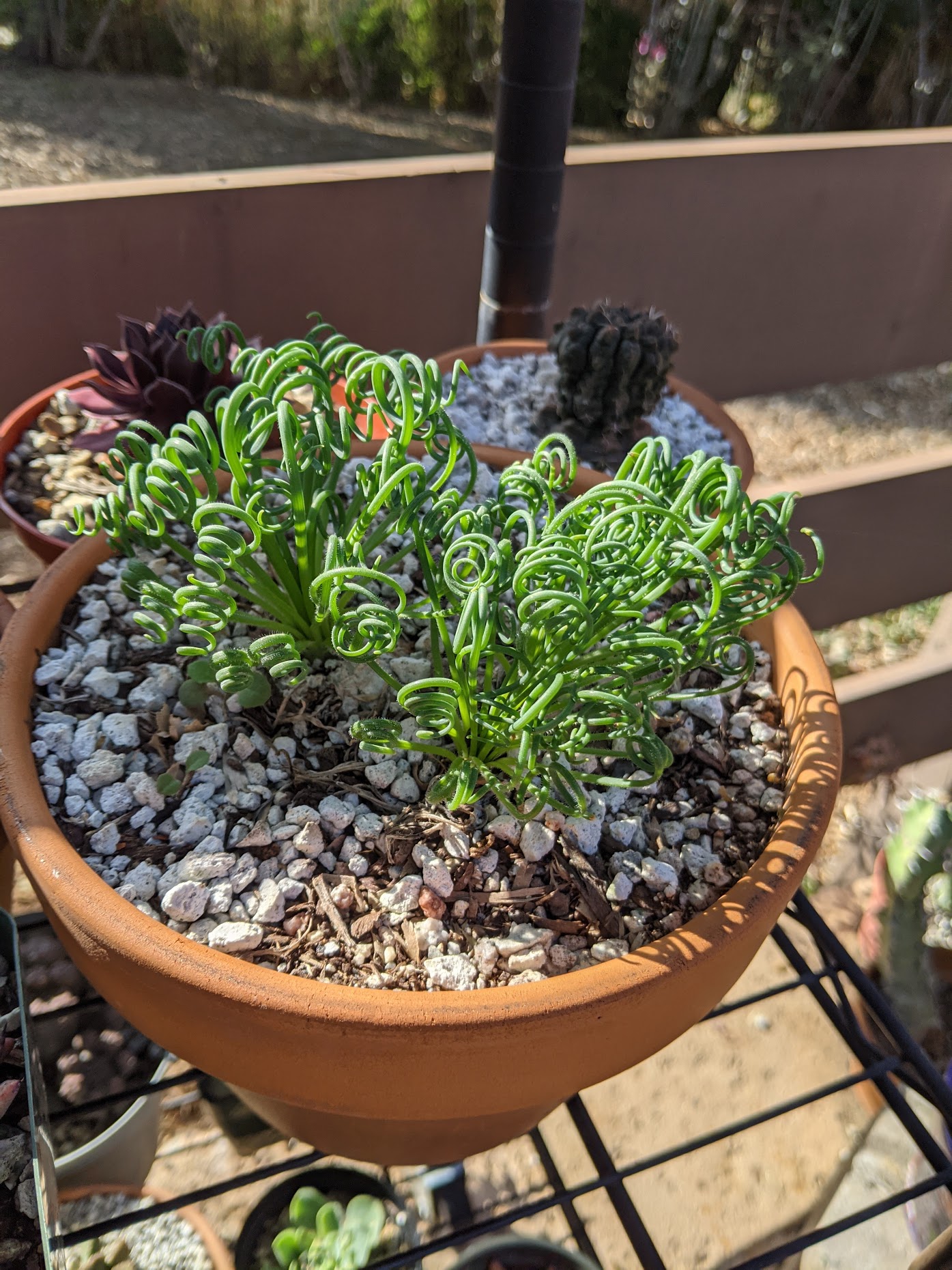The photograph is an outdoor close-up taken on a patio during the daytime. At the forefront, there is a large terracotta clay pot featuring green spiral-stalked plants, entwining and curling like green curly straws. These plants grow from a medium of small white or light gray rocks mixed with brown mulch. Just behind it, positioned slightly to the right, sits a smaller pot containing a stout round cactus, similarly rooted in gravel-strewn soil. To the left, another pot holds a red succulent, possibly a 'hen and chicks' plant. All three pots appear in the central focus, neatly arranged on a black wire plant rack. Additional potted plants can be seen beneath the rack, blurred slightly as they recede into the background. The setting is complemented by a wooden deck railing and faint glimpses of tree trunks and ground level elements, indicating that the photograph is likely taken on a deck elevated above a natural landscape.